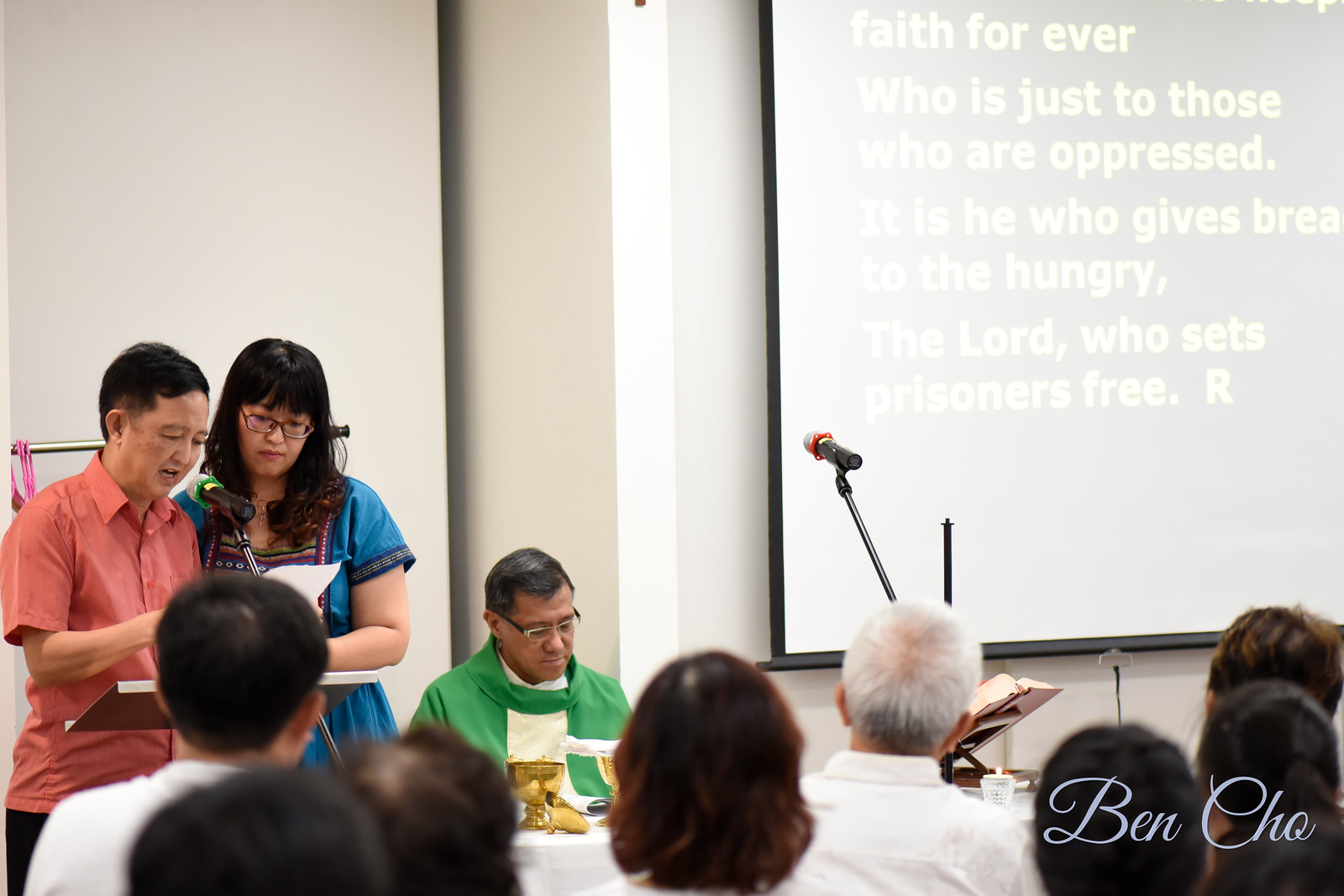In this detailed image of a church service, several elements stand out. In the foreground, the heads of congregants are visible, looking towards the front where the action is taking place. Taking that focus, on the left side at a podium, an Asian man is seen wearing a red button-down shirt, intently reading from a piece of paper. Beside him stands an Asian woman in a blue dress, also looking down at the same paper. In the background, a man dressed in a green religious garment is seated at a table, attention directed towards the podium. The center of the image features a microphone that remains unoccupied. In the top right corner, a projector screen displays text in sharp clarity against a white background. The text reads: "Faith Forever, who is just to those who are oppressed. It is he who gives bread to the hungry, the Lord who sets prisoners free." The color palette of the image is rich and varied, including shades of red, blue, green, pink, black, white, gray, brown, tan, orange, yellow, and gold. The setting is indoors, likely within a church or religious educational environment, with the atmosphere suggesting a religious presentation or service in progress.